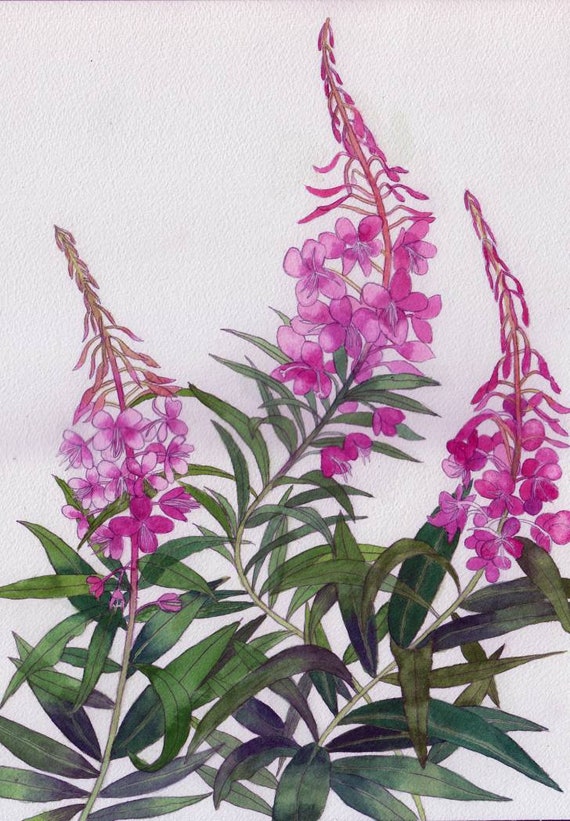This artwork is a stylized and attractive botanical drawing, potentially rendered in watercolor or colored pencil, featuring three pink flowers prominently displayed against a textured white background. The flowers, which are likely a variant of hyacinth or orchid, exhibit a captivating blend of bright fuchsia and pale pink hues. These blossoms grow vertically along light green stems, with expressive, thin, and wiry leaves that harmoniously intertwine. Each stem terminates in unopened buds shaped almost like arrows, indicating a blooming process that progresses from bottom to top. The foliage at the base consists of long, oval-shaped leaves in vibrant green tones accentuated by hints of purple and blue, adding depth and richness to the composition. This image captures the delicate and expressive nature of the flowers, emphasizing their potential for further growth and blossoming.